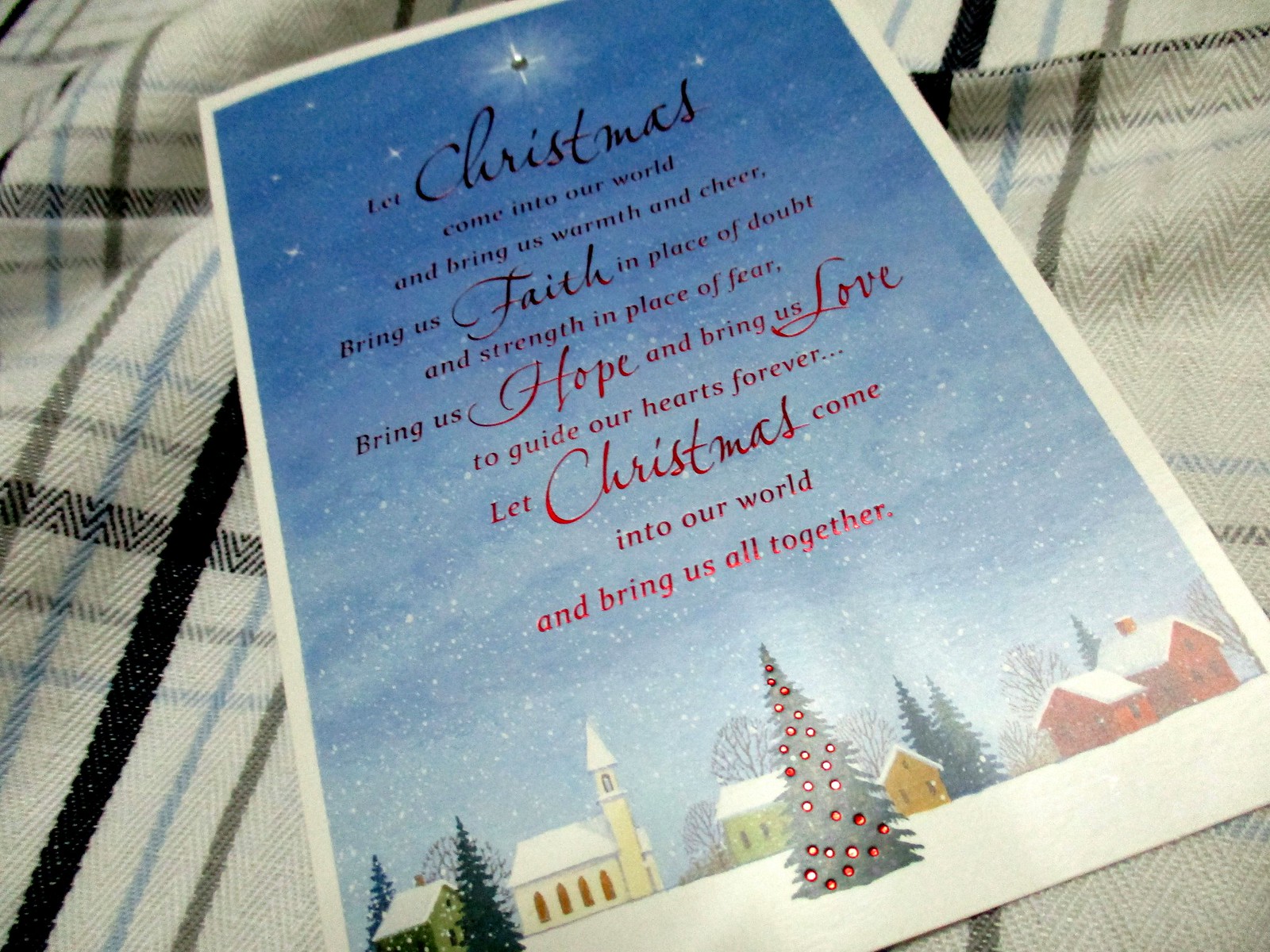The image captures an artistic Christmas card set at a diagonal on a plaid material, resembling a cozy blanket or scarf with a mix of white, black, blue, and green thin lines. The card itself features a snowy town scene with various small, colorful buildings including homes and barns at the bottom. Central in the scene is a decorated Christmas tree adorned with red ornaments. Above the town, the sky fades into a dark blue filled with stars and snowflakes. In elegant, shiny red font, the heartfelt text on the card reads: "Let Christmas come into our world and bring us warmth and cheer. Bring us faith in the place of doubt and strength in the place of fear. Bring us hope and bring us love to guide our hearts forever. Let Christmas come into our world and bring us all together."